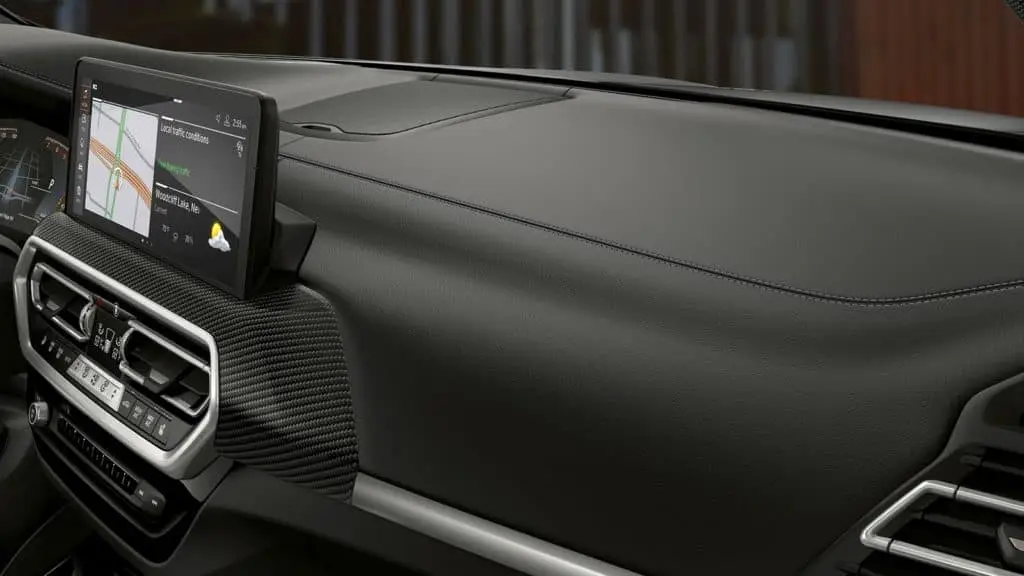In this image, we see a detailed view of a modern car's dashboard. The interior is predominantly black with silver or gray accents. The top portion of the image reveals the very bottom of the front windshield, with a blurred gray-lined area in front of it and a brown area to the right-hand side. 

The focal point is on the center console, where a touchscreen monitor is prominently featured. The screen displays a map on its left side, with a gray background, brown roadways, and a visible green line. To the right of the map, there is a graphic image showing a sun behind a cloud, along with various pieces of information in white and green text. The screen is framed in black and sits atop a broad area that includes two air vents outlined in silver or gray.

Below the screen and vents, there are multiple buttons, icons, and dials. The buttons in the center are gray, while those on the edges are black, all set within a black surface with more silver trimming. The area includes what appears to be radio controls and possibly a gas pedal further down. To the right of the center console, there is another air vent with silver lining, and the glove compartment features a silver bar, contributing to the sleek, modern aesthetic of the car's interior.